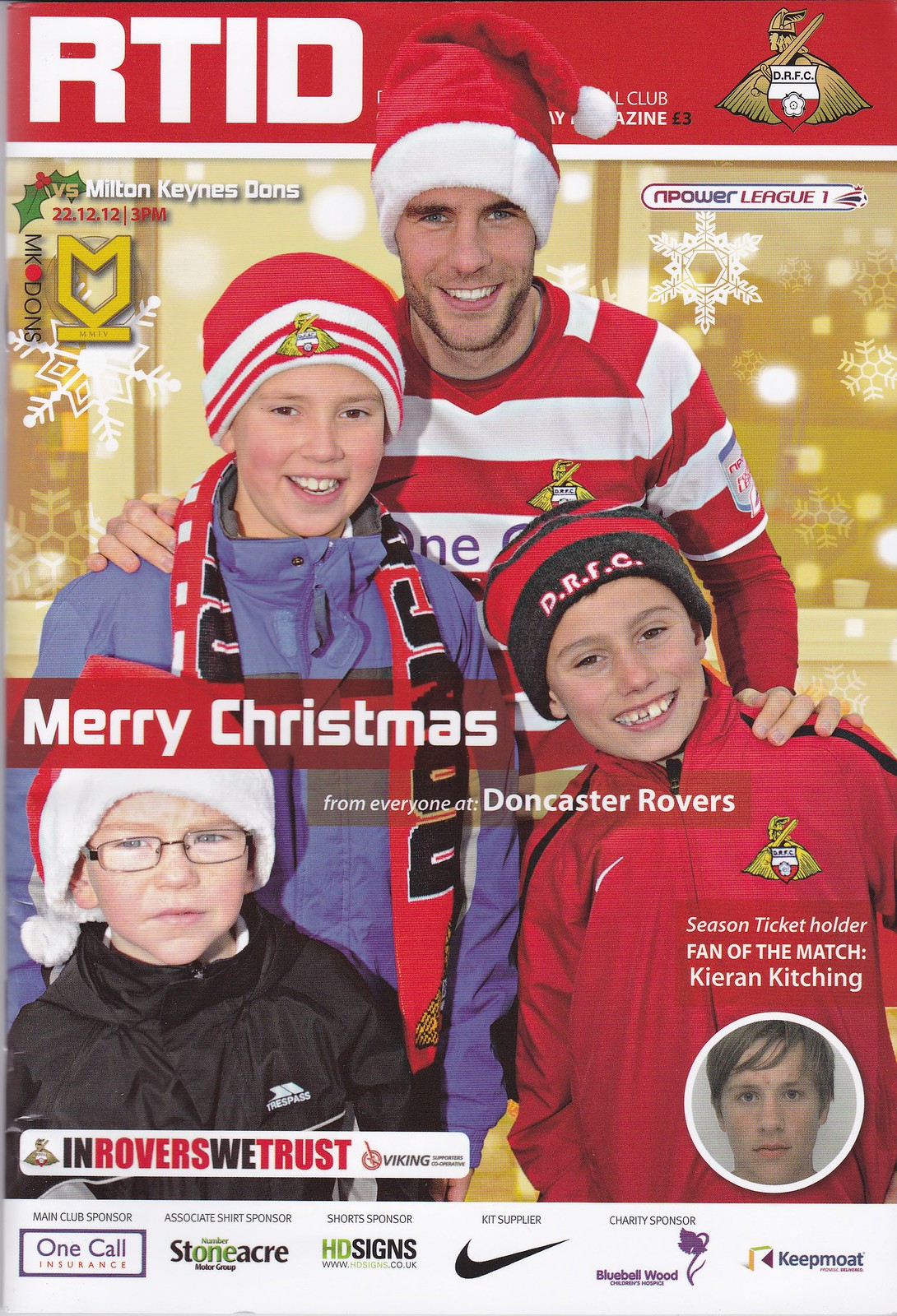This is a detailed description of an old magazine cover with a festive Christmas theme. At the top of the magazine, a prominent red bar with white lettering reads "RTID." The central feature of the cover is a photograph of a man, appearing to be around 35 years old, wearing a Santa hat with white trim. He is dressed in a horizontally striped red and white shirt and is smiling.

In the photo, the man has his hands on the shoulders of two boys standing in front of him. The shorter boy on the bottom right is light-skinned, smiling, and wearing a beanie hat. The caption next to him identifies him as "Season Ticket Holder Fan of the Match, Kieran Kitching." 

To the left of Kieran stands another boy, taller and wearing a red and white beanie hat, a blue jacket, and a red scarf. On the bottom left, a younger boy with glasses and a black coat is also wearing a Santa hat.

The background features a gold hue with snowflakes adding to the festive atmosphere. Over the center bottom of the photograph, white lettering spells out "Merry Christmas."

Additional elements on the cover include a small logo on the right side, depicting a Viking or knight with a sword, helmet, and cape, holding a shield that says "DRFC." On the left side, it lists "Versus Milton Keynes Dons, 22 12 12, 3 p.m," along with another logo. Below the main image, various logos for ads including One Call Insurance, Stoneacre Group, HD Signs, Nike, and Bluebell Wood Keepmoat are displayed. 

Overall, the cover sends warm holiday greetings from the Doncaster Rovers with cheerful imagery of fans and festive decor.